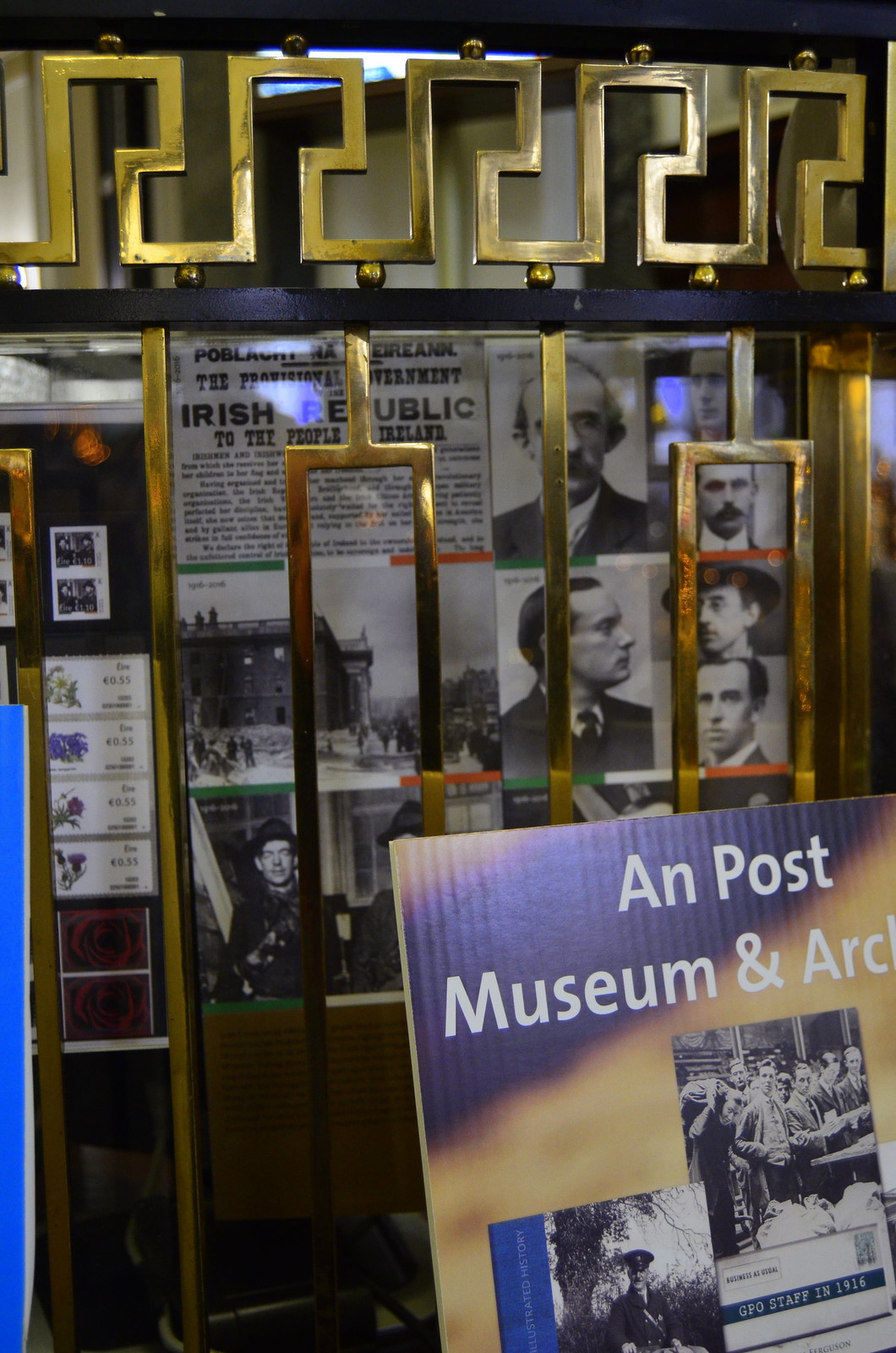The photograph depicts the front facade of the Ann Post Museum. Prominently featured is a golden and black iron gate with geometric designs, which stands in front of a sign. The top part of the sign partially visible reads "Ann Post Museum" with the remaining text cut off from view. Below this, black and white photographs are affixed to the sign. 

One of the photos, located on the bottom left, shows a man potentially in a police uniform. To the right of this is another black and white photograph of several men facing right. Behind the golden iron gate, there is a window displaying more black and white photographs, including newspaper clippings. A notable clipping reads "Irish Republic" with text above it that is partially obscured by light but appears to begin with "The Provisional Government" and continues below as "To the people of Ireland." The gate and the displayed images combine to create an intriguing view for museum visitors.